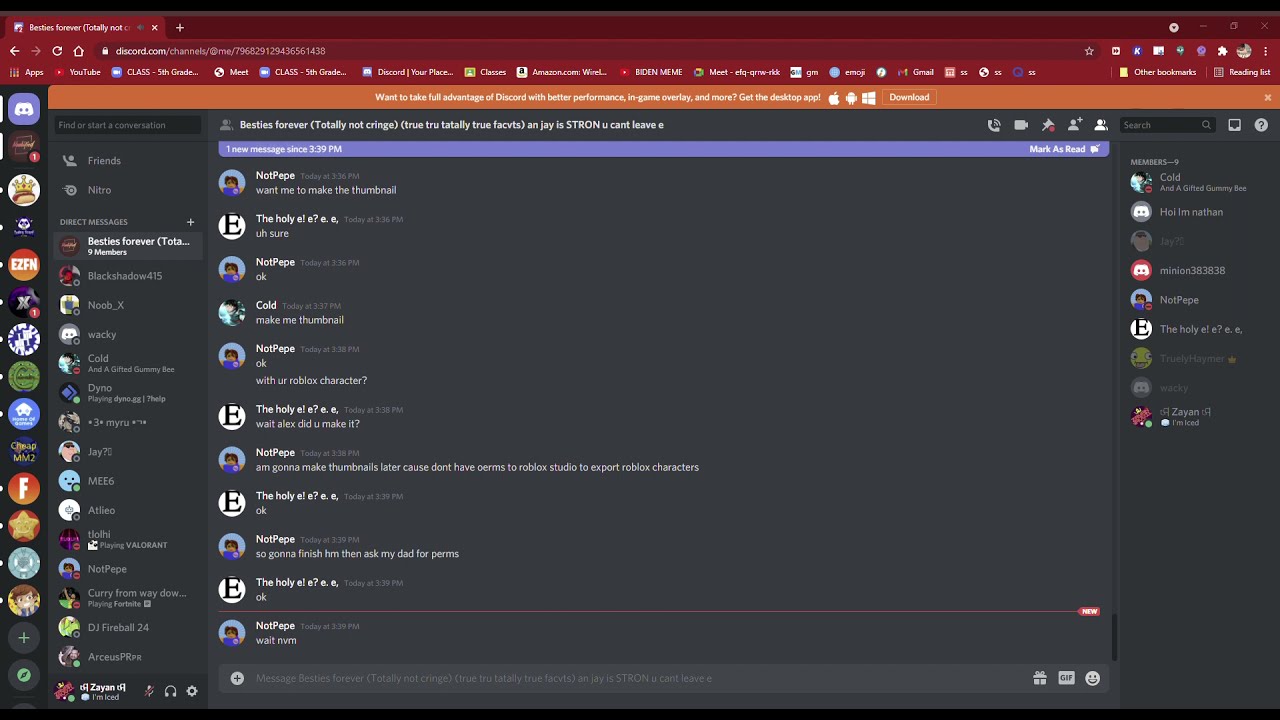The image is a detailed screenshot of a computer screen displaying a Discord webpage. The screen features a maroon bar at the top with a single open tab titled "besties forever totally not cringe." Underneath the search bar and across the top, there are numerous saved bookmarks for various apps, YouTube, Discord, Google Meet classes, Amazon, and a meme about Joe Biden, among others. 

The focal point of the image is a conversation between two users discussing the creation of a thumbnail featuring a Roblox character. The text exchanges are small and challenging to read but show back-and-forth messages: "Want me to make the thumbnail?" "Sure, okay." "Make me thumbnail, okay." "With your Roblox character?" and logistical details about permissions for Roblox Studio.

There are colorful icons and avatars throughout the screen, showcasing an array of colors such as black, white, gray, red, purple, orange, green, and yellow. Notable icons include YouTube, Discord, and an Amazon logo, alongside various other app icons and user avatars, such as a gold crown, a blue bear, and a kid with brown hair on a yellow background. The overall background is gray, adding to the dense and text-heavy nature of the screenshot. This image captures an active and visually packed digital environment centered around a Discord conversation.